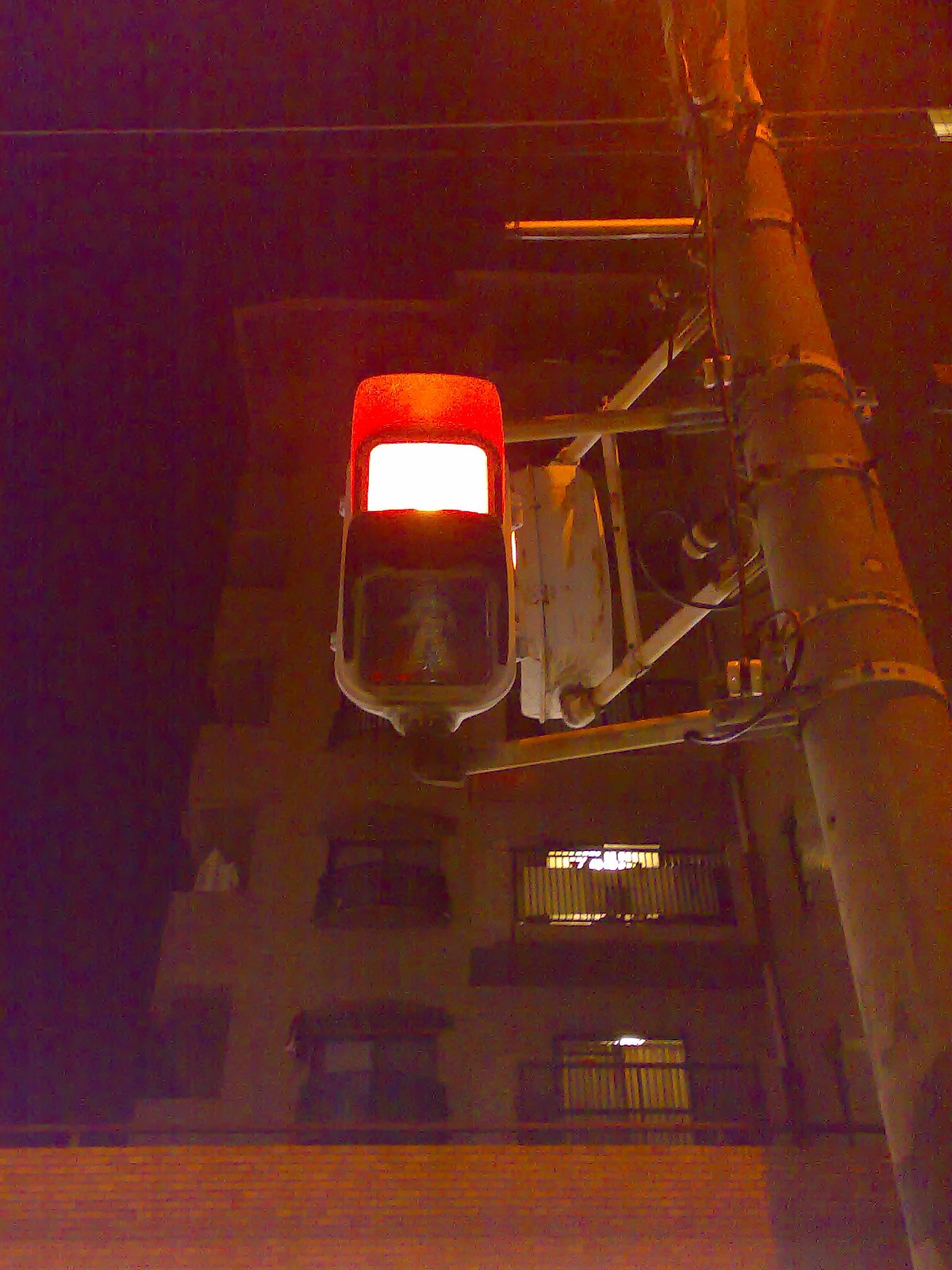The photograph captures a nighttime cityscape featuring a "Don't Walk" signal affixed to a pole, illuminated in bright red. Taken from a low vantage point, the signal is viewed from below, emphasizing its prominence. Behind the signal, the sky is inky black, emphasizing the late hour. A light brown apartment building with multiple windows and balconies rises in the background, providing a sense of urban density. The bottom of the image is framed by a brick wall, adding texture and a grounding element to the composition. The stark contrast between the illuminated signal and the dark surroundings draws attention to the importance of pedestrian safety even in the quiet of the night.